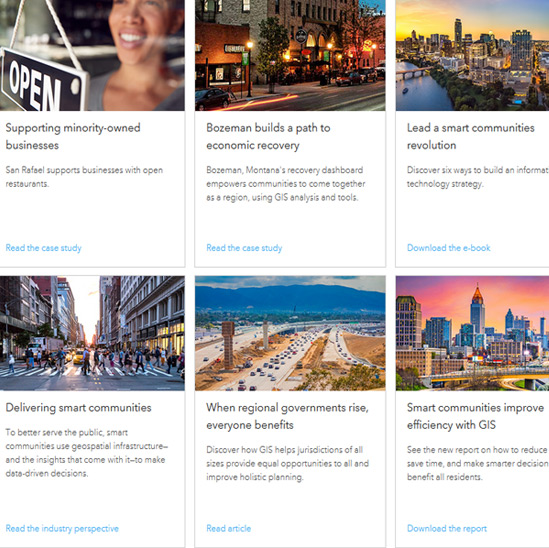Here is a detailed and cleaned-up caption for the described image:

---

The image is a grid featuring six thumbnails, arranged in a three-above-three block format, each corresponding to a news article about community and economic development initiatives. 

- **Upper Left:** A vibrant image of a young woman standing behind an 'Open for Business' sign. The caption reads, "Supporting Minority-Owned Businesses: San Rafael Promotes Open Restaurants." A link invites readers to "Read the Case Study."

- **Upper Center:** A nighttime photograph of a brightly lit storefront, accompanied by the text, "Bozeman Builds a Path to Economic Recovery." The subheading explains that Bozeman, Montana's recovery dashboard empowers communities to collaborate regionally using GIS analysis and tools. Readers are encouraged to "Read the Case Study."

- **Upper Right:** An aerial view of a city featuring a bridge spanning a river, captioned, "Lead a Smart Communities Revolution." The thumbnail advertises an article on "Six Ways to Build an Information Technology Strategy."

- **Lower Left:** A bustling urban scene with people crossing a street, headlined, "Delivering Smart Communities to Better Serve the Public." The description highlights how smart communities leverage geospatial infrastructure and insights to make data-driven decisions. A link directs readers to "Read the Industry Perspective."

- **Lower Center:** A scenic image of a highway cutting through a desert landscape with mountains in the distance. The caption, "When Regional Governments Rise, Everyone Benefits," promotes an article on how GIS helps various jurisdictions offer equal opportunities and improve holistic planning. The article is accessible via "Read the Case Study."

- **Lower Right:** A cityscape at sunset with the text, "Smart Communities Improve Efficiency with GIS." The accompanying description directs readers to a report on how GIS can streamline processes, save time, and enable smarter decision-making that benefits all residents.

---

This caption provides a detailed and structured description of the image, ensuring clarity and coherence.